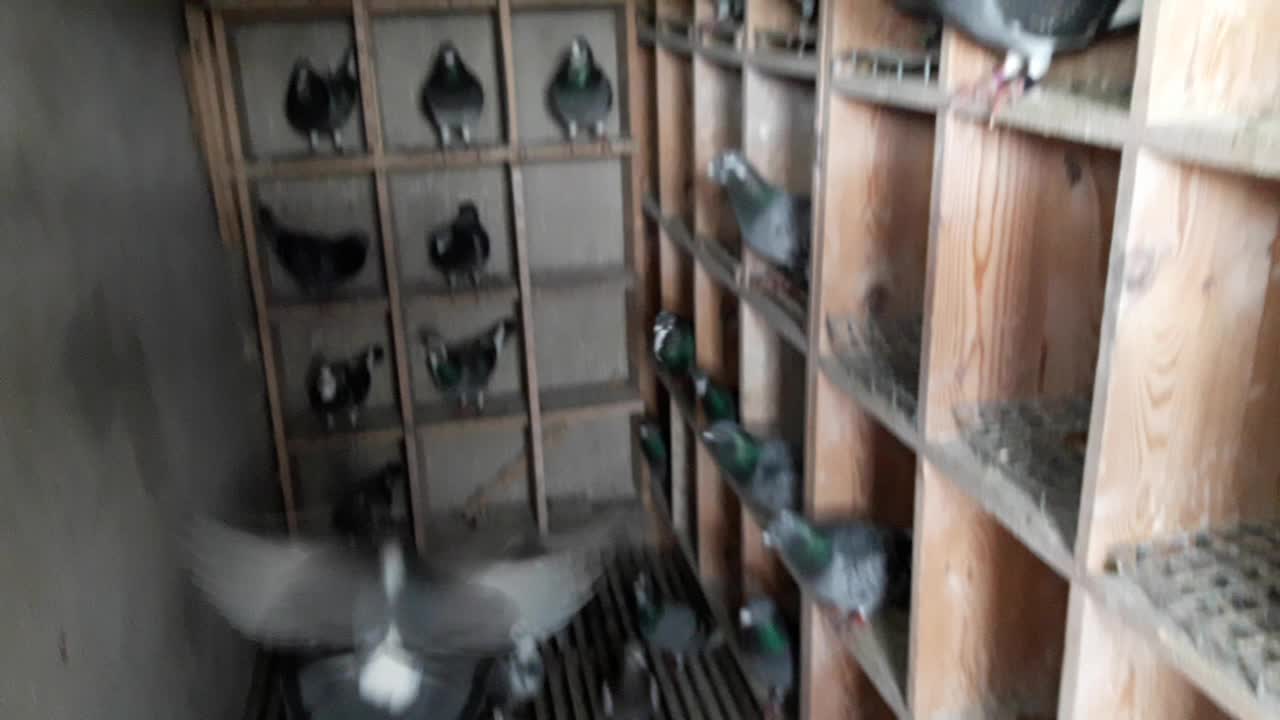The image is a blurry, close-up photograph of the interior of a pigeon coop, focusing on a densely populated roosting area. The coop is constructed from dimension lumber and features open-grid flooring. The back wall is lined with an array of roosting boxes, arranged in four rows of three, housing approximately nine pigeons, while the right wall has an additional set of roosting boxes sheltering around a dozen birds. Each pigeon is perched within these wooden boxes, which are filled with grating material. The foreground is dominated by a pigeon in mid-flight, its wings a blur of dark gray with lighter gray tips, and its body marked by a white head and tail base. The pigeons display variations in plumage, featuring gray feathers, white undersides, shiny green upper heads, and white beaks. The confined space and numerous birds contribute to an overall impression of a bustling, lively coop environment.